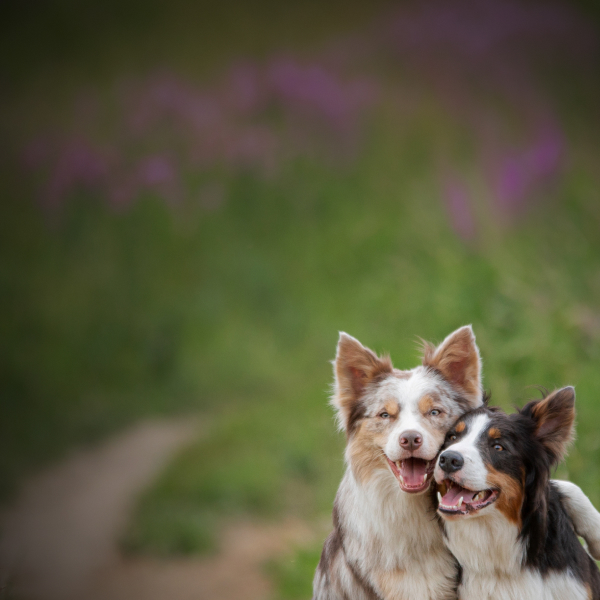In this charming photo, two exuberant Australian Shepherd mutts are cozily nestled together in the bottom right corner, sharply in focus against a beautifully blurred background. The backdrop is a vivid field of lush green grass and vibrant purple wildflowers, hinting at the natural beauty surrounding them. The dogs exude pure joy, their mouths open in wide smiles, and they sit with their faces touching, looking slightly left of the camera. One dog, predominantly black with tan and white markings, has his upper left leg lovingly draped around his companion, exhibiting a heartwarming bond. The other dog, with a marbled coat of white, light brown, and gray, leans in, both appearing content and thrilled to be outdoors. Three of their ears are perked up, with one ear playfully mashed against the other. This touching image captures the essence of their excitement, camaraderie, and the joyful simplicity of a sunny day in the field.